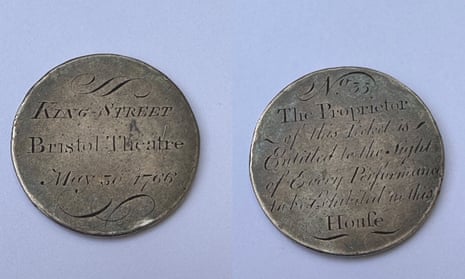This image features a close-up shot of a vintage, round silver coin, prominently positioned against a blue background. Displaying both front and back views, the coin appears to serve as an entry ticket to a theater performance. On the left side of the coin, an inscription reads, "King Street, Bristol Theatre, May 30th, 1776." The right side bears the number "35" accompanied by a scripted note indicating, although partially faded, that the ticket grants the proprietor entry to a performance. The metal surface of the coin is dark gray and shows signs of wear, with the lettering and inscriptions significantly faded, giving it an antique appearance.